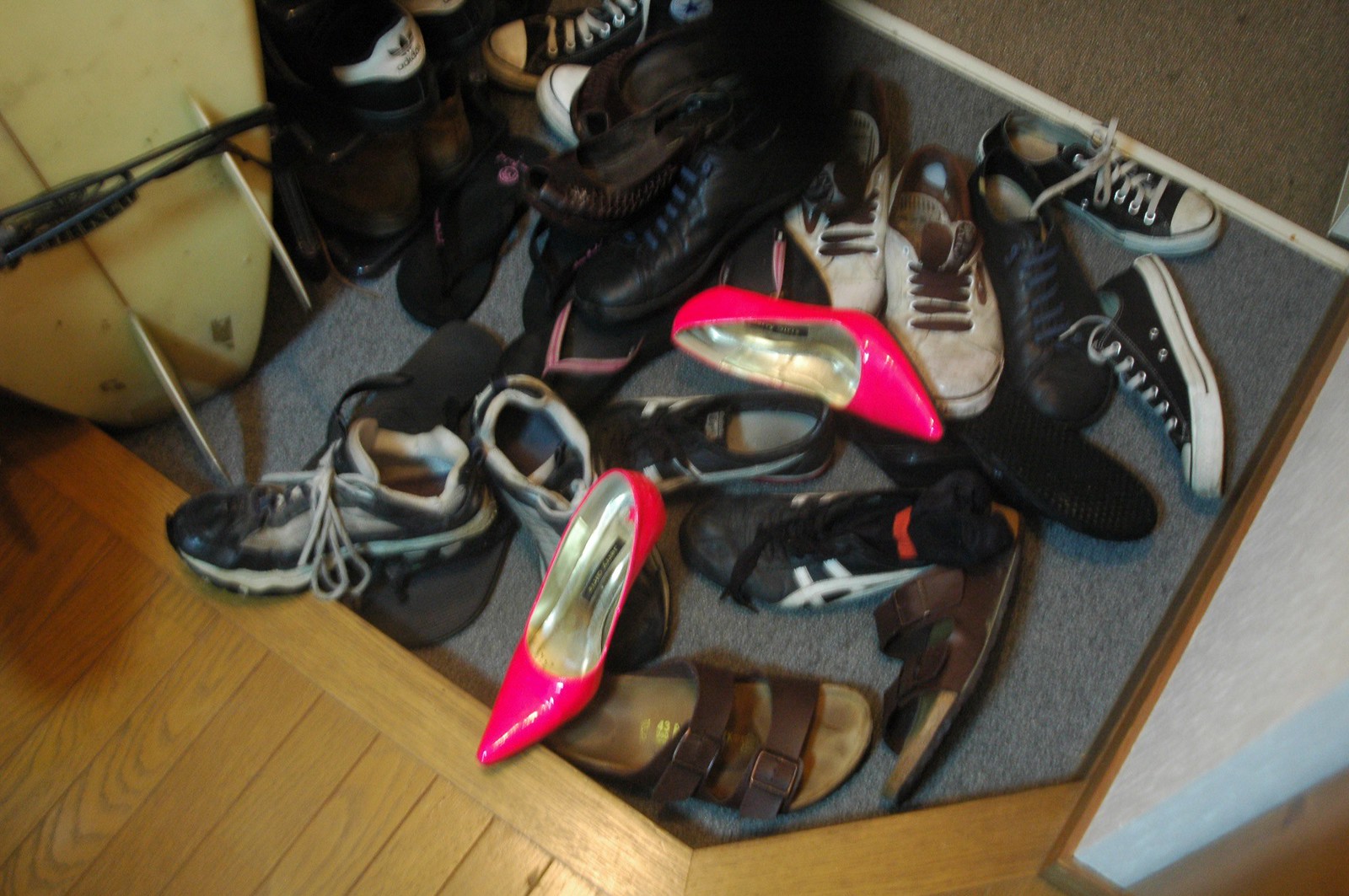The image displays a cluttered assortment of over 12 pairs of shoes, jumbled together on a gray carpet laid over a wooden floor. The collection includes various types of footwear, predominantly sneakers in colors like black, white, blue, and brown. A pair of shiny pink pumps with pointed toes and a silver interior stand out prominently. Also visible are pink-topped black slippers, brown leather sandals, and black and white Adidas sneakers with distinct logos. To the left, a vertical surfboard leans against the wall. Additionally, there's a brown timber frame at the bottom right and a brown object with a black frame and silver legs in the top left corner of the image.